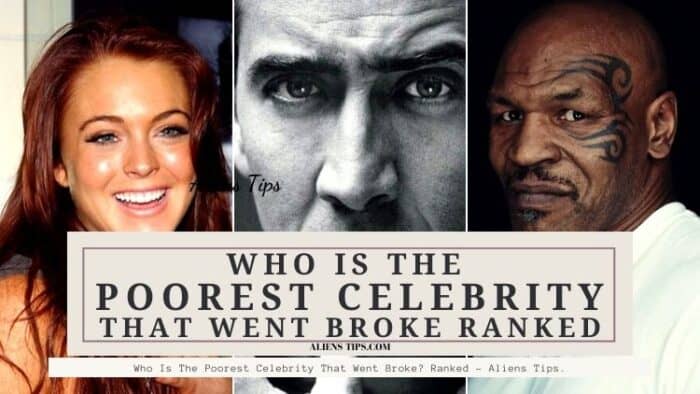The image is a landscape-oriented composition divided into three vertical sections featuring prominent celebrities. On the left is Lindsay Lohan, smiling warmly into the camera with her distinct long, reddish-brown hair framing her face, although her outfit remains obscured by a label. The middle section showcases a black and white photograph of Nicolas Cage, exuding a familiar actor's charisma. To the right, Mike Tyson is depicted with his recognizable bald head and a distinctive curved tattoo pattern around his left eye, complemented by a thin mustache and goatee, as he stares directly into the camera. Overlaying the bottom of the image is a large white rectangle bordered in gray, containing bold black text that reads, "Who is the poor celebrity that went broke ranked?" Below this, in smaller text, the source is identified as "alientips.com."